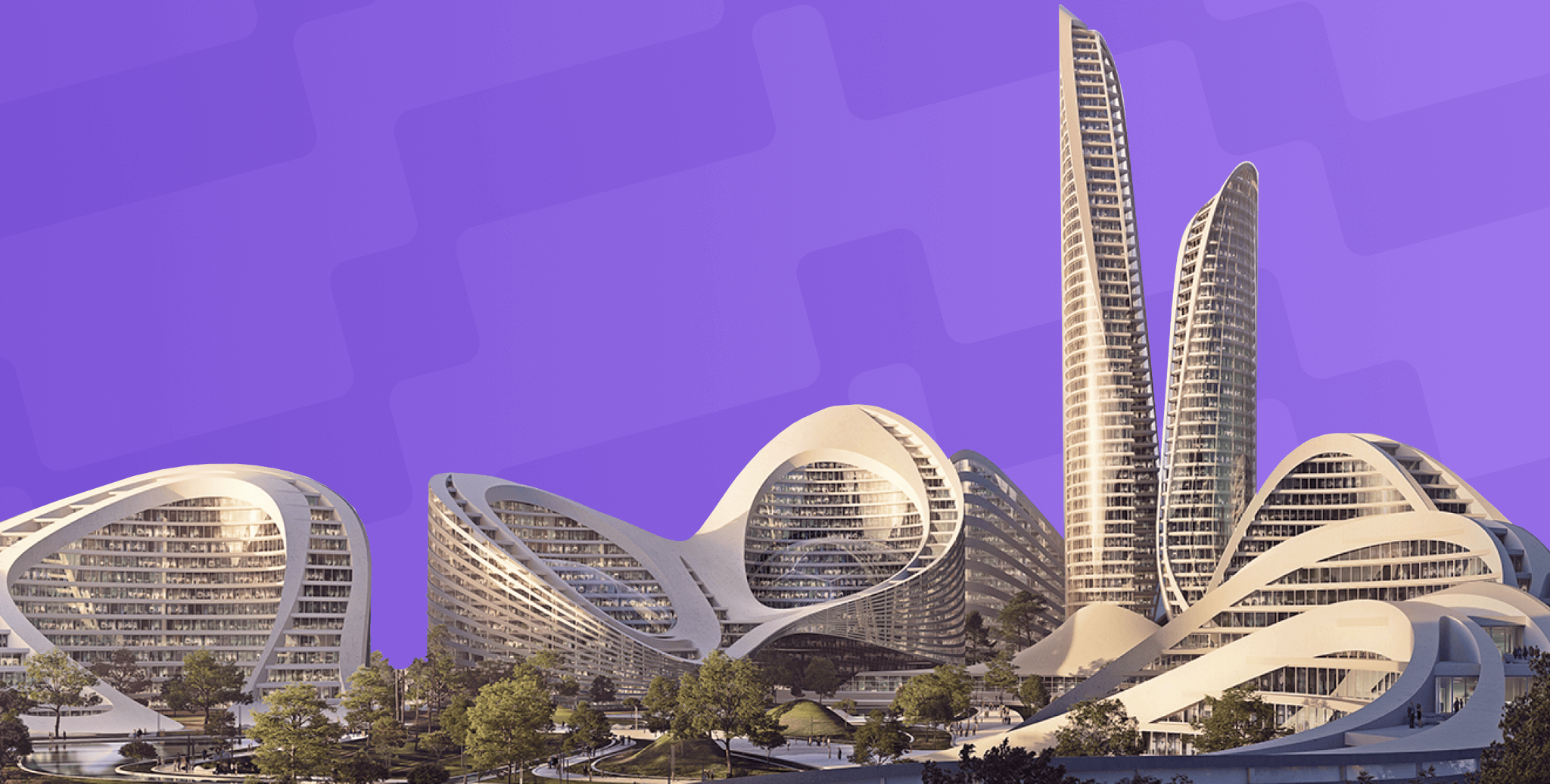The image depicts an architect's detailed rendition of a futuristic modern city complex. Central to the image are various white and gray buildings with avant-garde designs, including vertical skyscrapers, spiraled structures, and horizontal constructs adorned with numerous windows. These buildings are artistically shaped to appear like waves, giving them a dynamic and fluid appearance. The foreground features lush green trees, wide sidewalks, and people walking around patio and asphalt areas, adding a layer of serene, everyday life to the scene. The background is a striking composition of purples and blues, textured to create a vibrant yet harmonious backdrop to the sleek, metallic-looking constructions. The overall impression is one of a highly sophisticated and futuristic urban landscape.